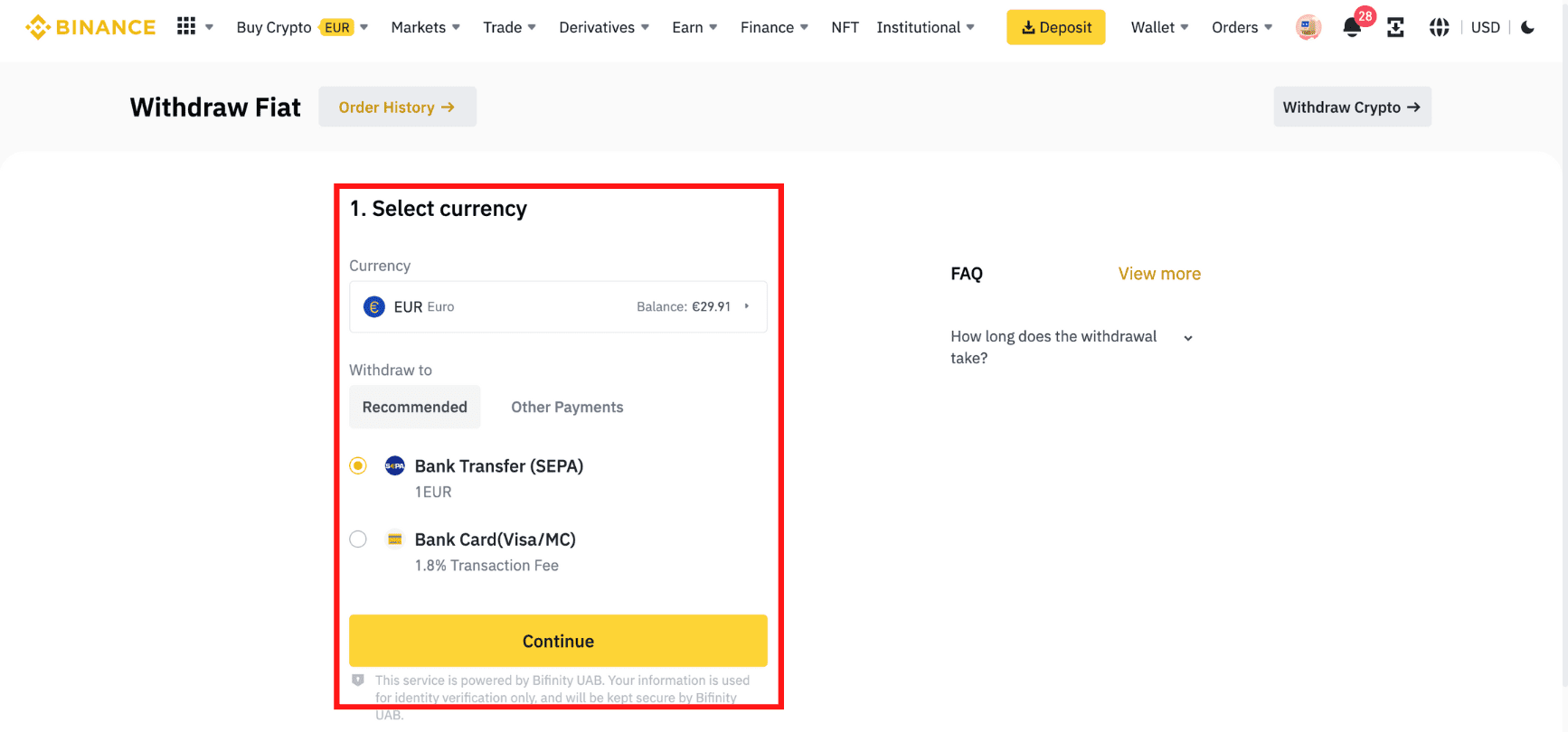This is a detailed screenshot of the Binance dashboard, a platform associated with cryptocurrency and finance. The image has a white background that seamlessly blends with the interface, giving a clean and uncluttered look. In the upper left-hand corner, the Binance logo is prominently displayed in yellow. Several drop-down menus are situated next to the logo, including options like Buy Crypto, with EUR selected in a gold oval, indicating European currency. Other menu items include Markets, Trade, Derivatives, Earn, Finance, NFT, Institutional, Deposit, Wallet, and Orders. Additional user icons provide functionalities such as Notifications and Withdraw Fiat. 

On the right-hand side, there's a dedicated button for Withdrawing Crypto. Below this, a box surrounded by a red border on the left side is labeled Select Currency. Currently, EUR (Euros) is selected with a balance displayed as 29.91 EUR. The box also includes options for withdrawing currency, specifying that at the moment, a Bank Transfer via SEPA is selected for a fee of 1 EUR.